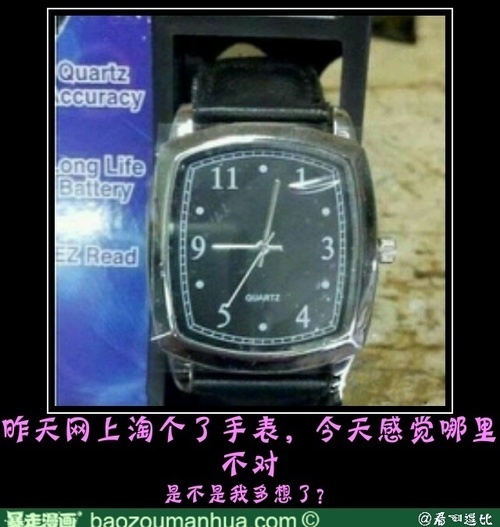A square advertisement image featuring a somewhat blurry photograph of an unusual watch occupies the center. The watch face, which has a silver bezel and a black band, displays atypical numeral positions: where the number 7 would usually be is a 5; the numbers around the watch face are 1, 3, 4, 5, 9, and 11, with dots indicating the remaining positions. The watch hands point to approximately 9:02. To the left of the watch photo, a blue strip highlights key features: "Quartz Accuracy," "Long Life Battery," and "Easy Read." Beneath the watch image, a section of purple text in an Asian language is visible, followed by a green strip below it containing additional Asian text with a website address. The bottom right corner of the image features white graphics or logos against the background.